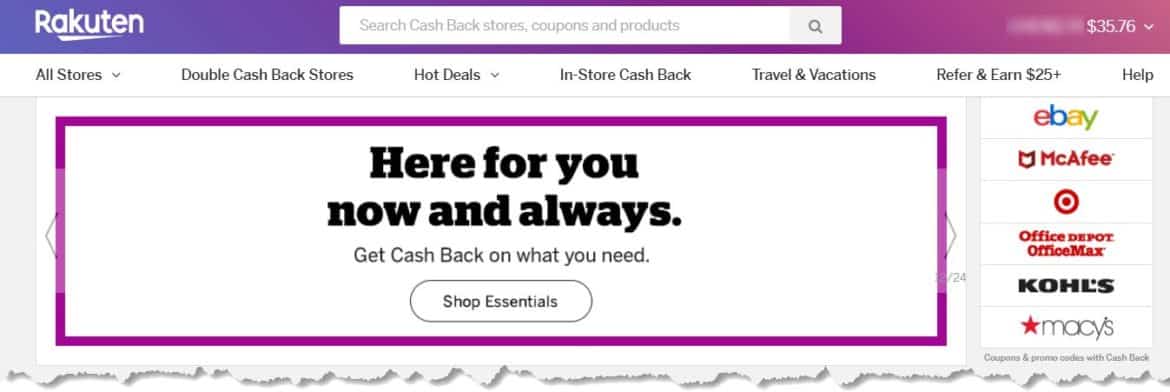This is a stylized screenshot from the Rakuten website, as identified by the prominently placed Rakuten logo in the upper left-hand corner. The logo, rendered in white, stands against a banner showcasing a striking gradient transitioning from blue to purple to pink from left to right. The header of the site features a search bar with a grayed-out search icon. Inside the search bar, light gray placeholder text reads, "Search Castback Stores, Coupons, and Products." 

In the upper right-hand corner, there is a username displayed in a subtle blue tone, alongside a monetary amount of $35.76 and a drop-down arrow, suggesting user earnings or account balance. Below this, the site's navigation bar offers various options: "All Stores" with an accompanying drop-down arrow, "Double Cashback Stores," "Hot Deals" with another drop-down arrow, "In-Store Cashback," "Travel and Vacations," "Refer and Earn $25+," and "Help."

The main content area of the page features an image carousel, equipped with faint left and right arrows for navigation. The prominently displayed image within the carousel conveys the message, "Here for You Now and Always," followed by, "Get Cashback on What You Need," and a "Shop Essentials" button encouraging user interaction. To the right of the carousel, a curated list showcases various stores and products, including notable names like eBay, McAfee, and Target, among others.